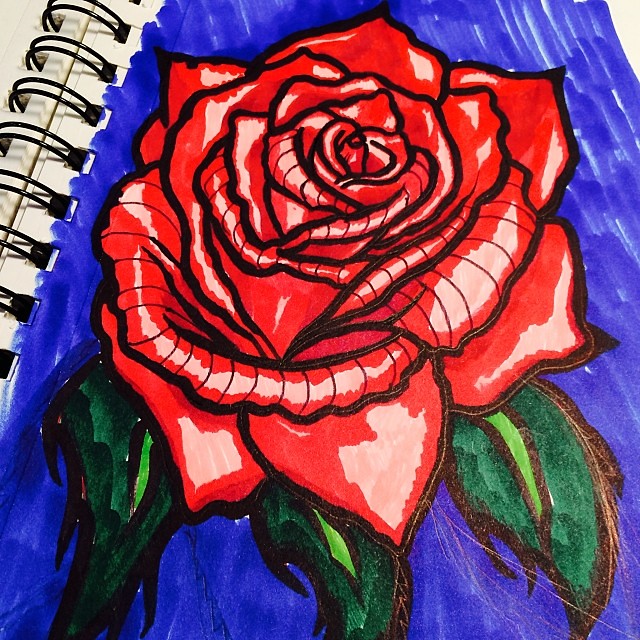In this vivid drawing captured within an art spiral ring book, the black, sturdy rings securely encircle pristine white paper. At the heart of the artwork is an exquisite close-up of a rose, depicted with meticulous attention to detail. The rose, nearly fully bloomed, exhibits a complex layering of six to ten petals, beginning with a tightly clustered center that gradually unfurls into more expansive outer petals. 

Three dark green leaves, each featuring lighter green centers, elegantly drape down from the bottom of the flower. The artist has skillfully employed thick, dark marker lines to define the edges, while finer lines, possibly from a thin-point marker, introduce intricate detailing within the petals. 

The rose petals predominantly boast a rich red hue. However, the artist has thoughtfully left sections of the petals white, suggesting a deliberate two-tone effect that adds depth and dimension. Subtle hints of pink in these white areas further enhance the delicacy of the floral portrayal. 

Surrounding this vibrant rose, the background is filled in with a medium blue, creating a striking contrast that makes the flower stand out. The entire composition is a testament to the artist's ability to combine bold colors with fine details, crafting a piece that is both vivid and profoundly engaging.